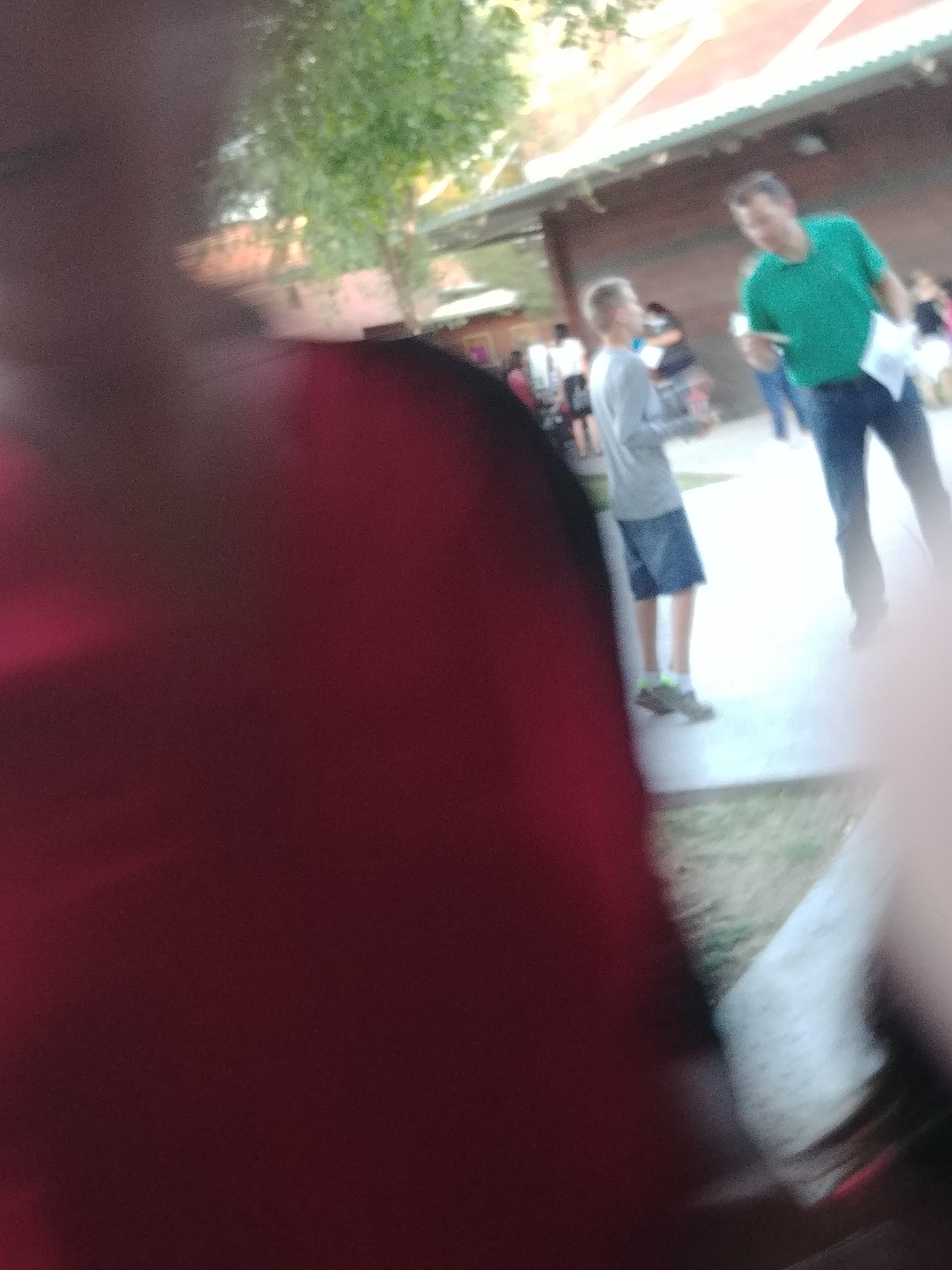The photograph is an outdoor scene taken in what appears to be a park or school yard. The image is very blurry in the foreground, dominated by an indistinct person wearing a red shirt with black stripes on the sleeves. This person occupies much of the picture and obscures finer details of their appearance. Beyond this person and slightly to the left, the background becomes clearer: a young boy, who is Caucasian and dressed in a gray long-sleeved shirt, jean shorts, and tennis shoes, is on his tiptoes engaging with an older man. The man, also Caucasian, is wearing a green collared shirt and blue jeans, and appears to be pointing at something or holding a piece of paper. Behind them, a concrete walkway stretches out, with other people scattered around a wooden or brick building. Leafy green trees frame the scene, suggesting a casual, relaxed atmosphere where people are gathered and interacting.